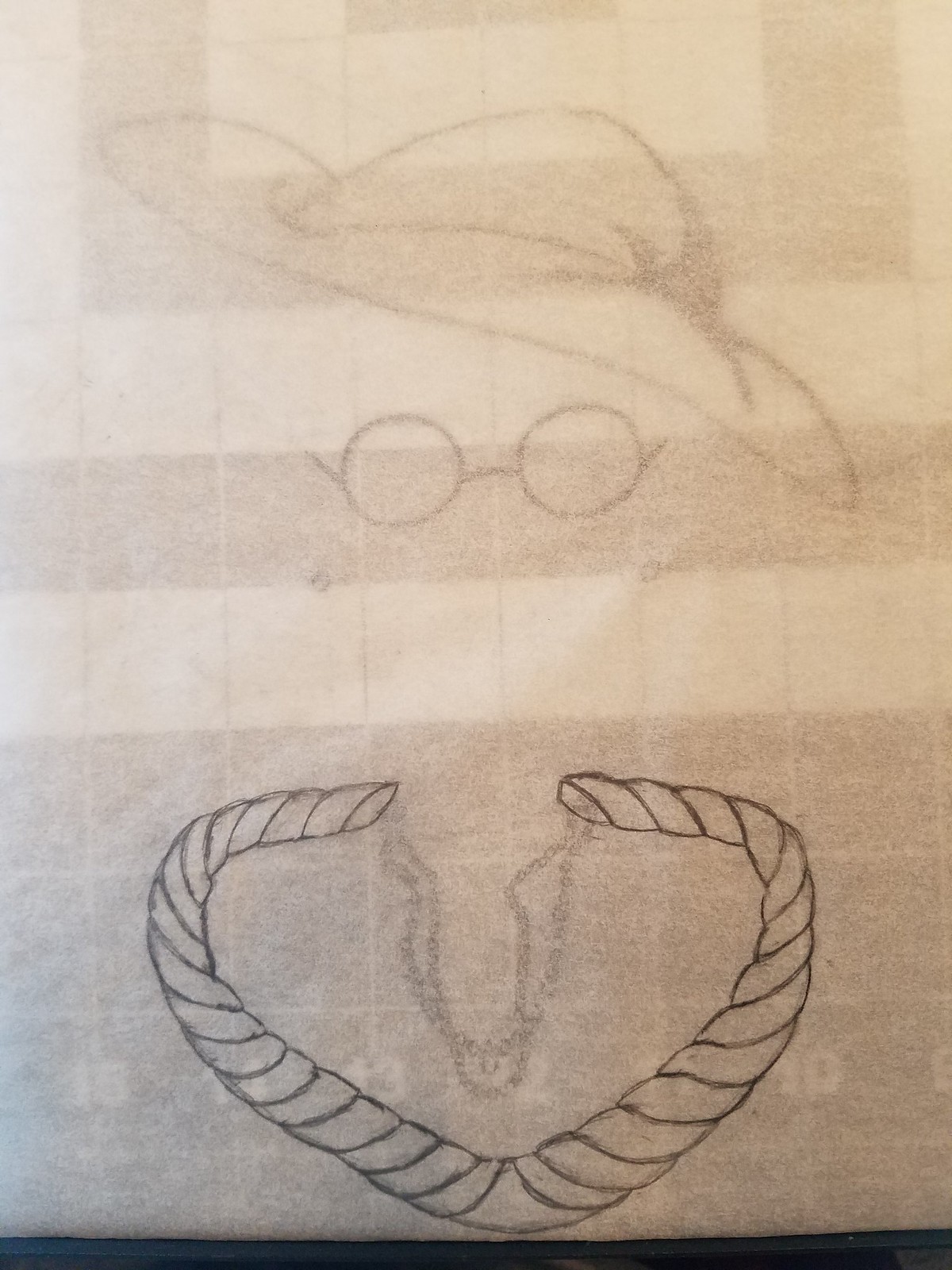This image features a delicate sketch rendered on an exceedingly thin, almost transparent piece of paper, allowing a charming quilt beneath to show through. The quilt's design is discernible, with a quilt square positioned at the top of the image, followed by a quilted border, and another quilt square at the bottom. The sketch itself, drawn with a light touch of pencil, depicts a woman's hat. The hat, characterized by its wide brim, angles gently upwards towards the left, while its rounded crown leans rightward. Notably, the sketch lacks a face, showcasing only a pair of round eyeglasses. Completing the drawing is an intricately twisted neckline or a type of rope-like adornment at the bottom.